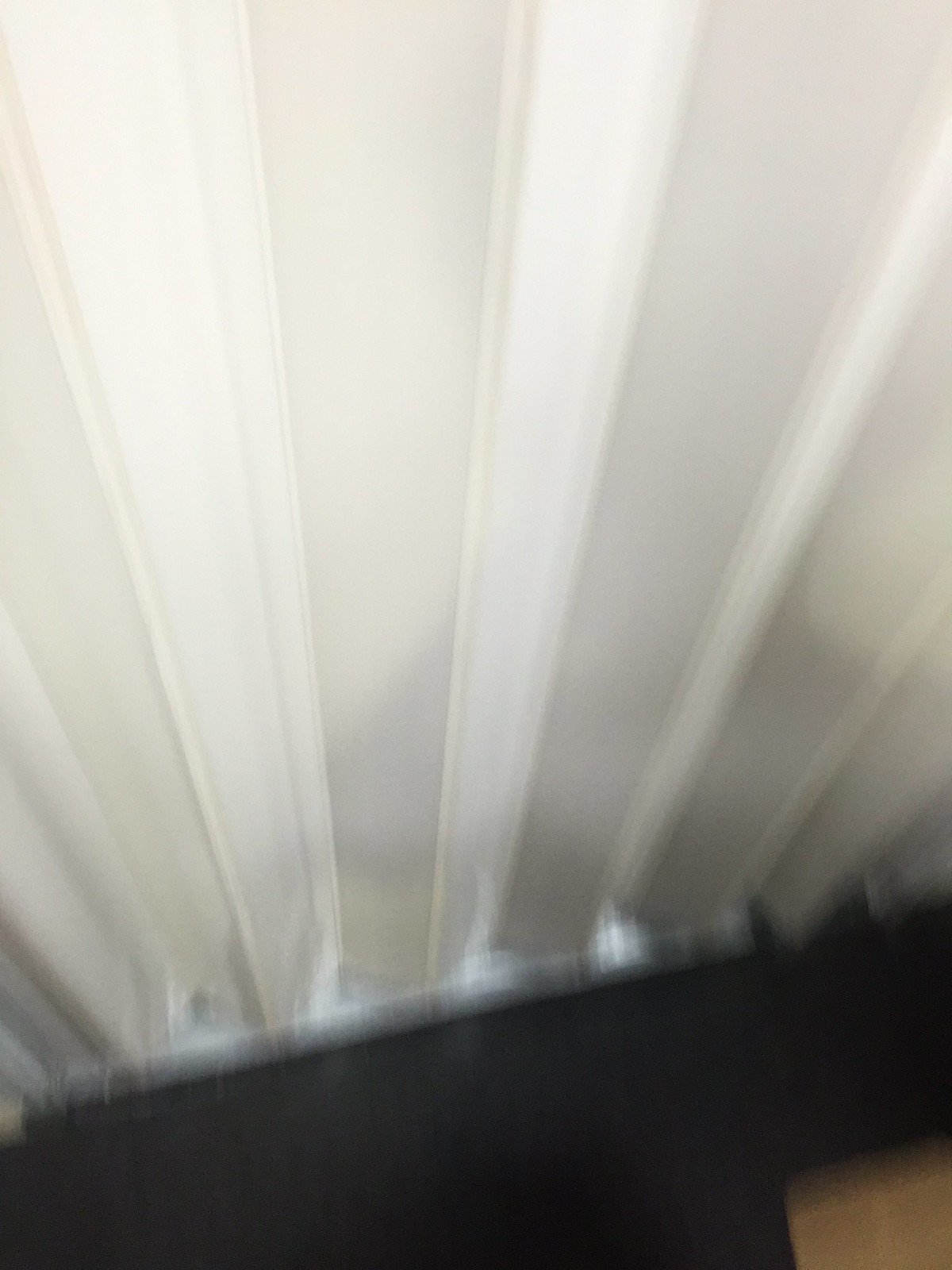In this blurry image, a prominently white object with vertical grooves and a corrugated texture dominates the frame. This structure appears ribbed and metallic, resembling the kind of material often found on the walls of a storage or shipping container, or potentially a steel shed. Along the bottom, there is a solid, silver-colored metal base. Both the grooves and the base run vertically from top to bottom. Stark contrasts are evident with black areas, which include a diagonal black strip at the bottom left corner about an inch up, widening to two inches on the right-hand side. The lower right corner contains a small section of lighter wood tone flooring. Additionally, atop this black region, shadows are cast on a white, slatted ceiling, enhancing the image's depth. Some darker white and lighter white slats create contrast. Shadows obscure further details, rendering some aspects indistinct, but possibly hinting at a glossy painted finish.